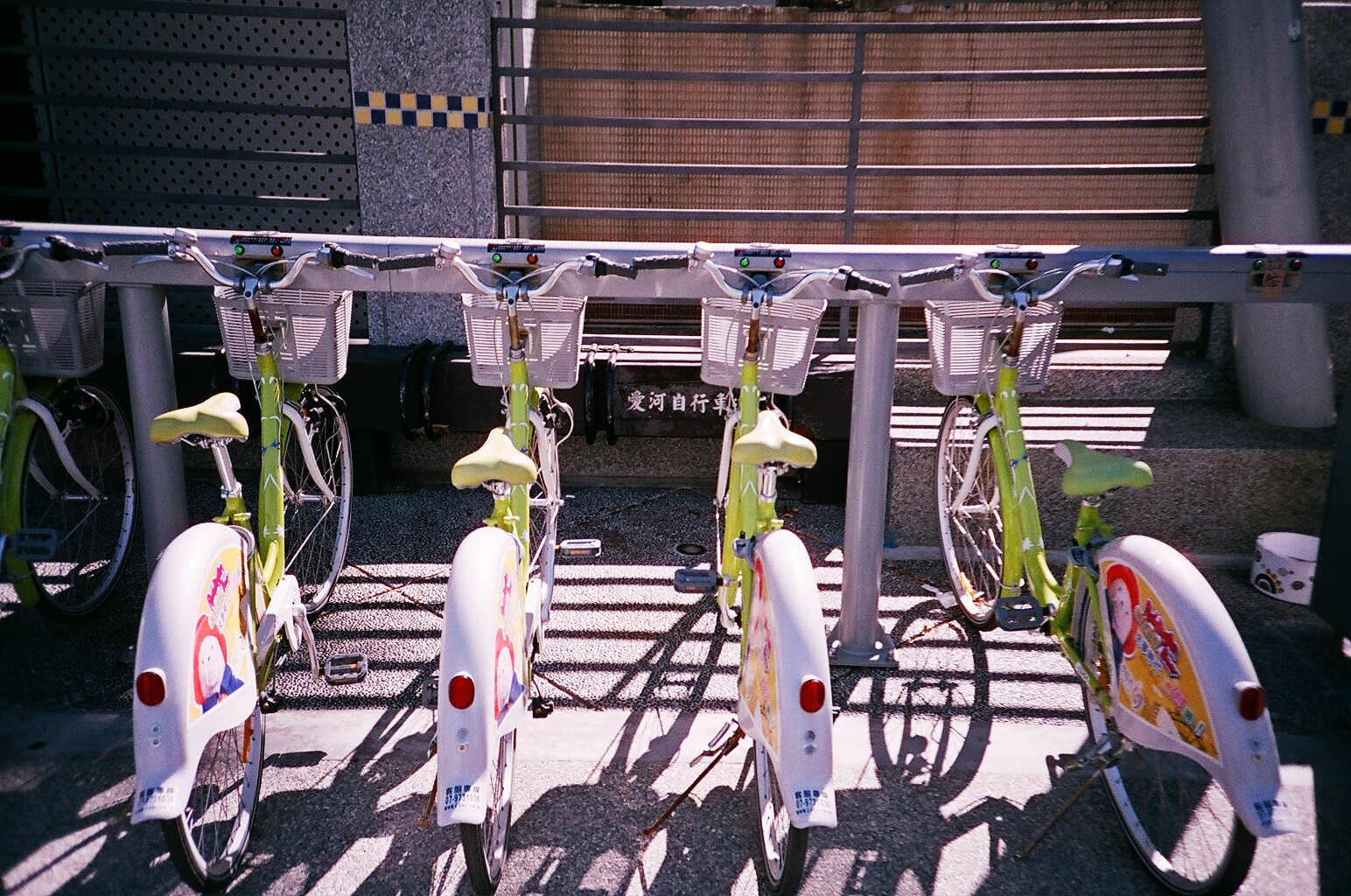The photograph captures a row of five lime green bicycles parked at a docking station, possibly in Japan, as suggested by the Japanese characters on a black pipe or construction piece in the background. The bikes, which may be electronic due to the visible green and red indicator lights on their docking stations, are neatly lined up with their back wheels facing the camera, revealing white wheel covers adorned with a cartoon image and additional writing. Each bicycle features distinct white baskets at the front, silver metal handlebars with black grips, and a white back wheel cover with a centered red light. The docking station includes control panels for rentals, suggesting a system where users can rent the bikes by paying or swiping a card. The backdrop of the image includes a wall and a metal grated gate.